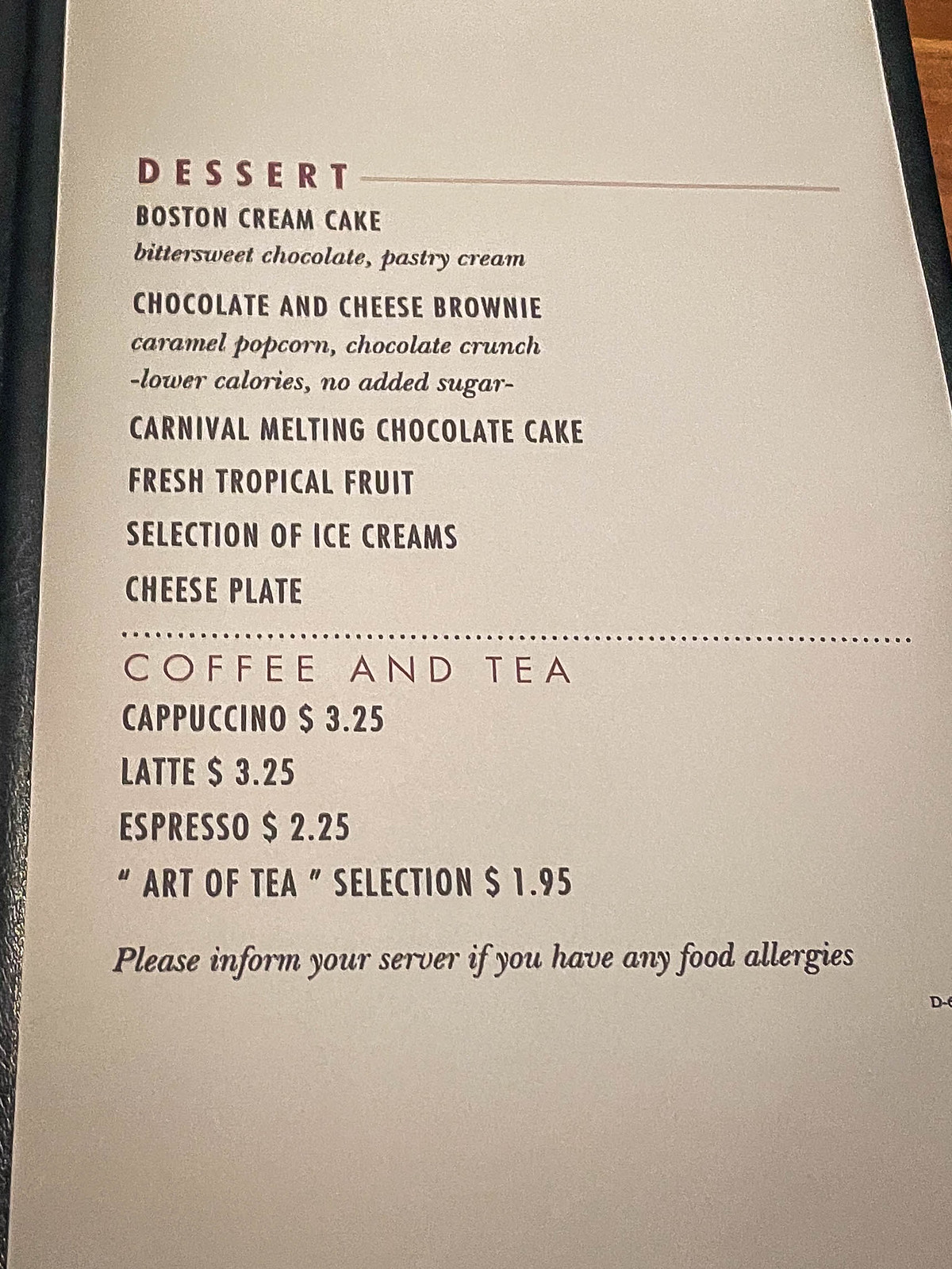**Image Caption:**
A detailed view of a menu at a restaurant or food stall. The menu has a vertical layout with a white background at the top. In bold, red, capitalized sans serif letters, the word "DESSERT" stands out, followed by a horizontal line extending halfway up the "T" to the right.

Below, in black, capitalized text, the menu lists the following desserts:
- Boston Cream Cake
- Bittersweet Chocolate and Pastry Cream
- Chocolate and Cheese Brownie
- Caramel Popcorn
- Chocolate Crunch (labeled as lower calories and no added sugar)
- Carnival Melting Chocolate Cake
- Fresh Tropical Fruit
- Selection of Ice Creams
- Cheese Plate

A dotted line separates this section from the beverages.

In a modern sans serif, capitalized font, it lists:
**Coffee and Tea**
- Cappuccino $3.25
- Latte $3.25
- Espresso $2.25
- Art of Tea Selection $1.95